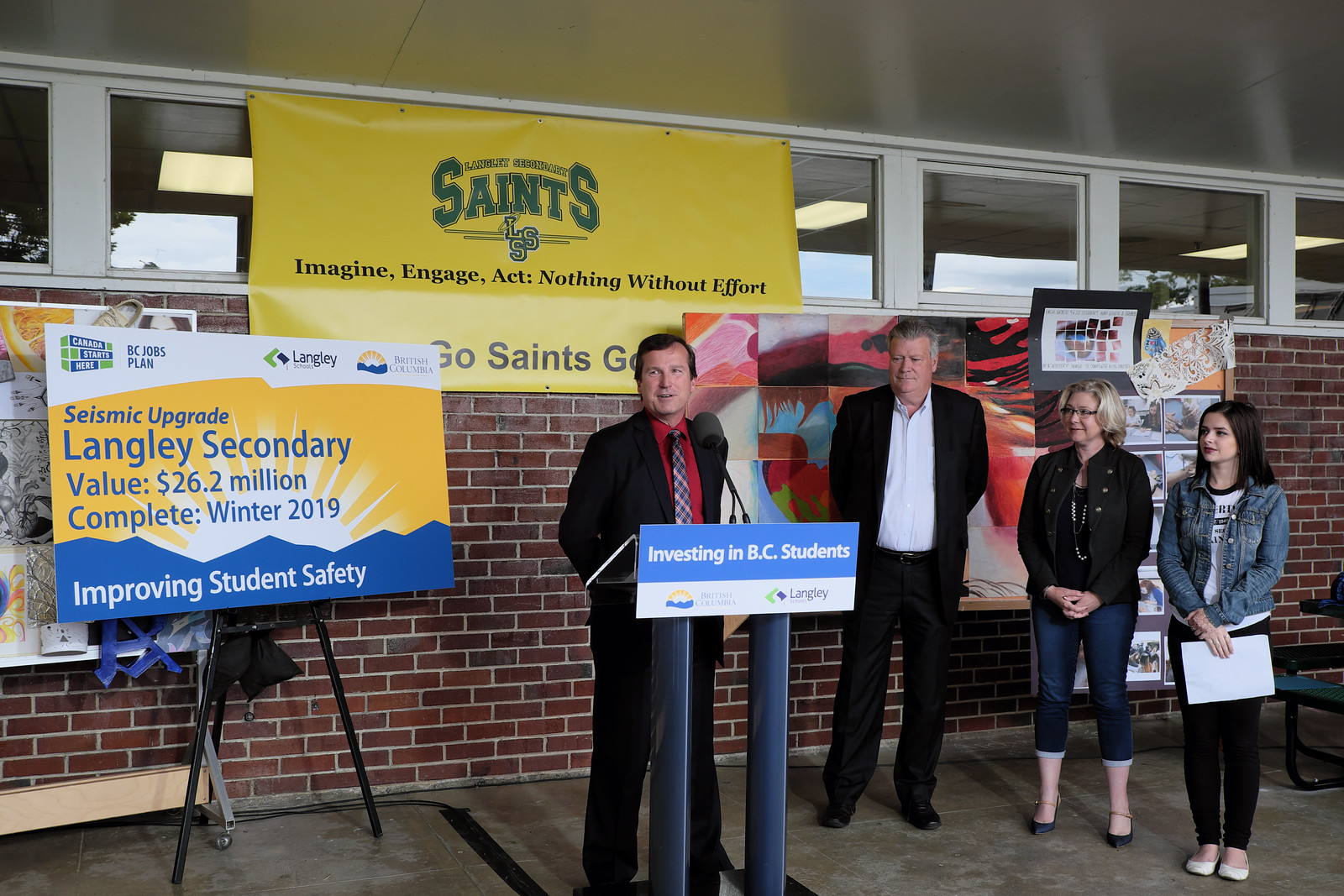In front of a brick wall and a banner that reads "Langley Secondary Saints, Imagine, Engage, Act, Nothing Without Effort, Go Saints Go!," a group of individuals is poised for an outdoor press conference highlighting efforts to enhance student safety. The focal point of the scene is a man in a black suit, red dress shirt, and black and gold tie standing behind a podium labeled "Investing in BC Students." Behind him are three attentive individuals—a man in a black suit and white shirt, flanked by two women—all seemingly prepared to speak. To their left, a tripod supports a detailed sign proclaiming the project's scope: "Seismic Upgrade, Langley Secondary, Value $26.2 million, Complete Winter 2019," emphasizing the improvement of student safety. The setting, rich with school pride and symbolism, depicts a concerted community effort to invest in and protect the local students.